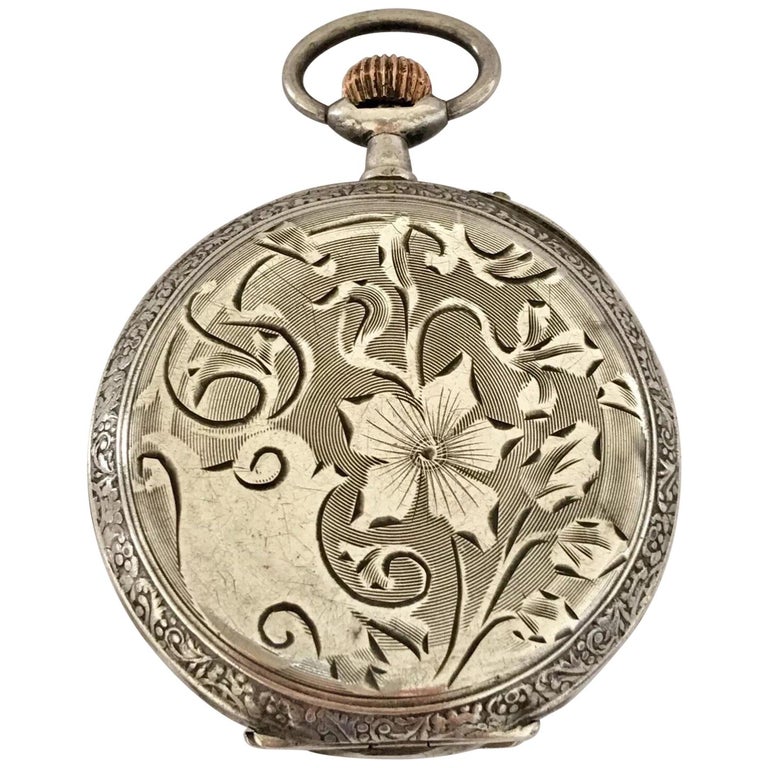The image showcases an extreme close-up of a closed, silver pocket watch, set against a pure white background that draws attention to its intricate design, potentially suggesting it is an item for sale. The antique watch appears to be in relatively good condition, with a polished surface that bears slight scratches over the detailed engravings. 

The lid of the pocket watch is adorned with an ornate engraving: a central flower with five petals is encircled by a vine motif, and this floral pattern extends into the surrounding filigree work that embellishes the perimeter. This filigree design is characterized by fine line work that emphasizes the motion and texture of the leaves and vines.

At the top of the watch, a crown-shaped winding mechanism is connected to a wide circular ring, allowing the watch to be worn on a chain. The hinge, visible at the bottom, indicates where the watch would open. The overall design and structure suggest it is an antique piece, possibly an Eastern Asian inspired locket or pendant, given its decorative elements and functionality.